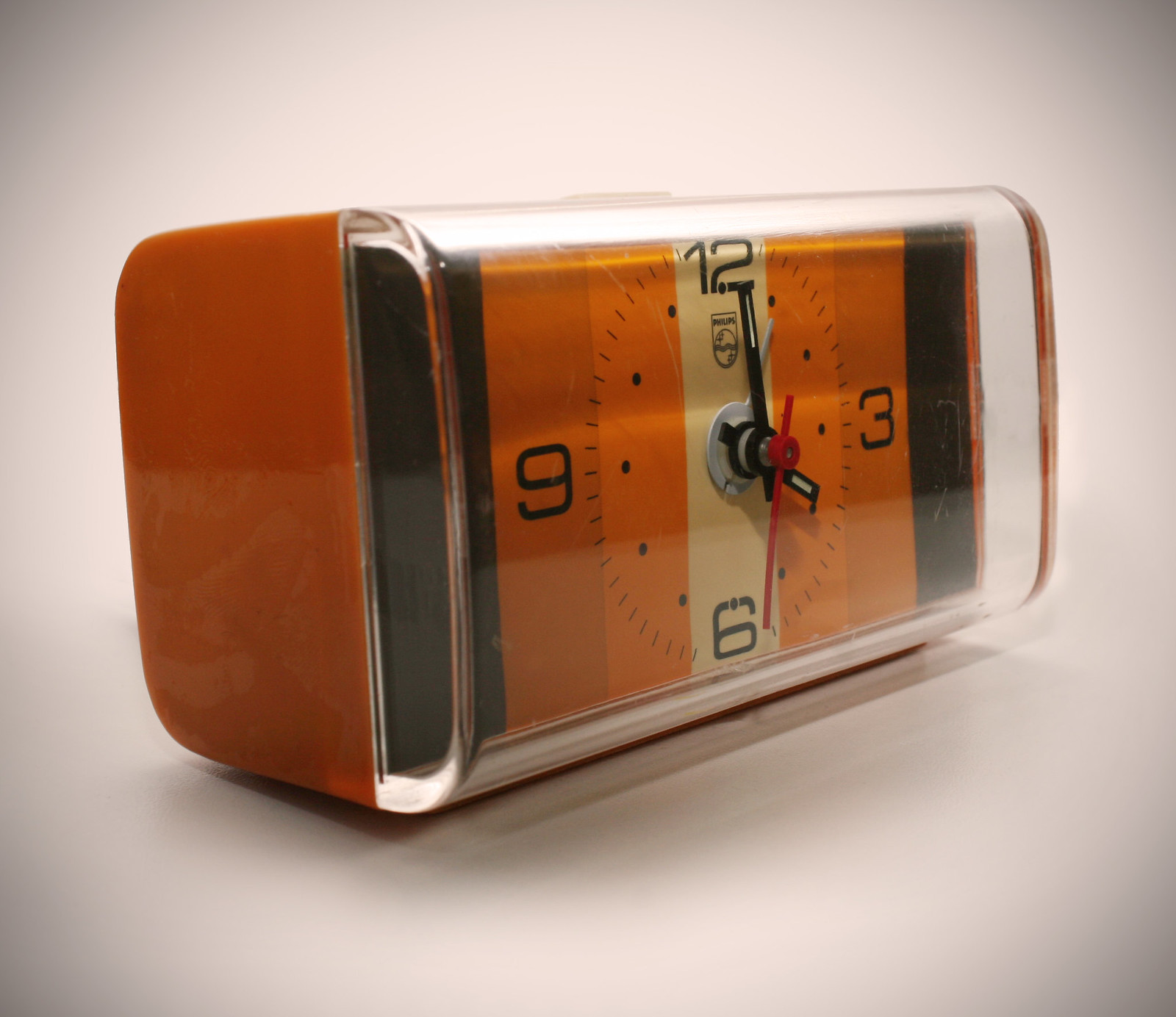This square-shaped image features a solitary clock set against a pristine white background. The clock itself is rectangular with an orange border, and it features a transparent glass front. The clock's face is visually striking, with a mix of colors: an outer ring of orange, a band of dark orange, and a central white section. A black rim encircles the clock face, adding depth and contrast. Uniquely, the clock displays only four numerals—12, 3, 6, and 9—arranged in a counterclockwise fashion, contributing to its distinctive appearance.